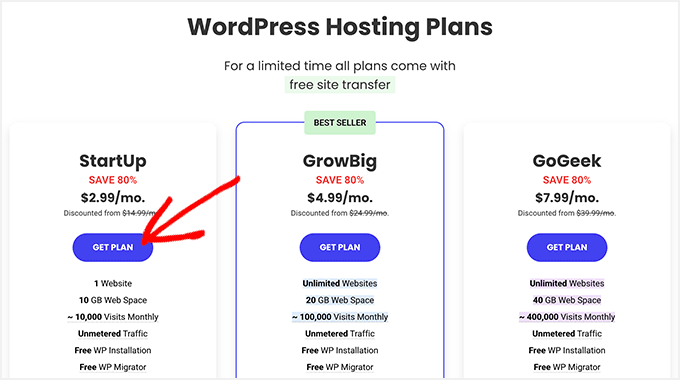The image caption has been refined and detailed as follows:

---

At the top, in bold black text, it reads "WordPress Hosting Plans." Beneath this text, a promotional note states, "For a limited time, all plans come with free site transfer," with a light green background highlighting the "free site transfer" portion. 

To the left, in black text, the first plan is described: "Startup" with an 80% discount, now priced at $2.99 per month, displayed next to a purple circle containing the text "Get Plan." An arrow, seemingly added via an editing program, points right from the "Get Plan" circle.

In the center, the term "Bestseller" appears atop a green background. Below this, the "GrowBig" plan is detailed: "Save 80% - $4.99 per month" (discounted from its original price of $24.99 per month, with a strikethrough).

An arrow extends from "Bestseller" pointing left to the "Get Plan" option for this package.

Lastly, the "GoGeek" plan is described to the right, stating "Save 80% - $7.99 per month," (discounted from its original price of $39.99 per month, with a strikethrough), alongside a purple "Get Plan" option. Below this, key features are listed against a light purple background: "Unlimited websites, 40GB web space, and 400,000 visits monthly."

---